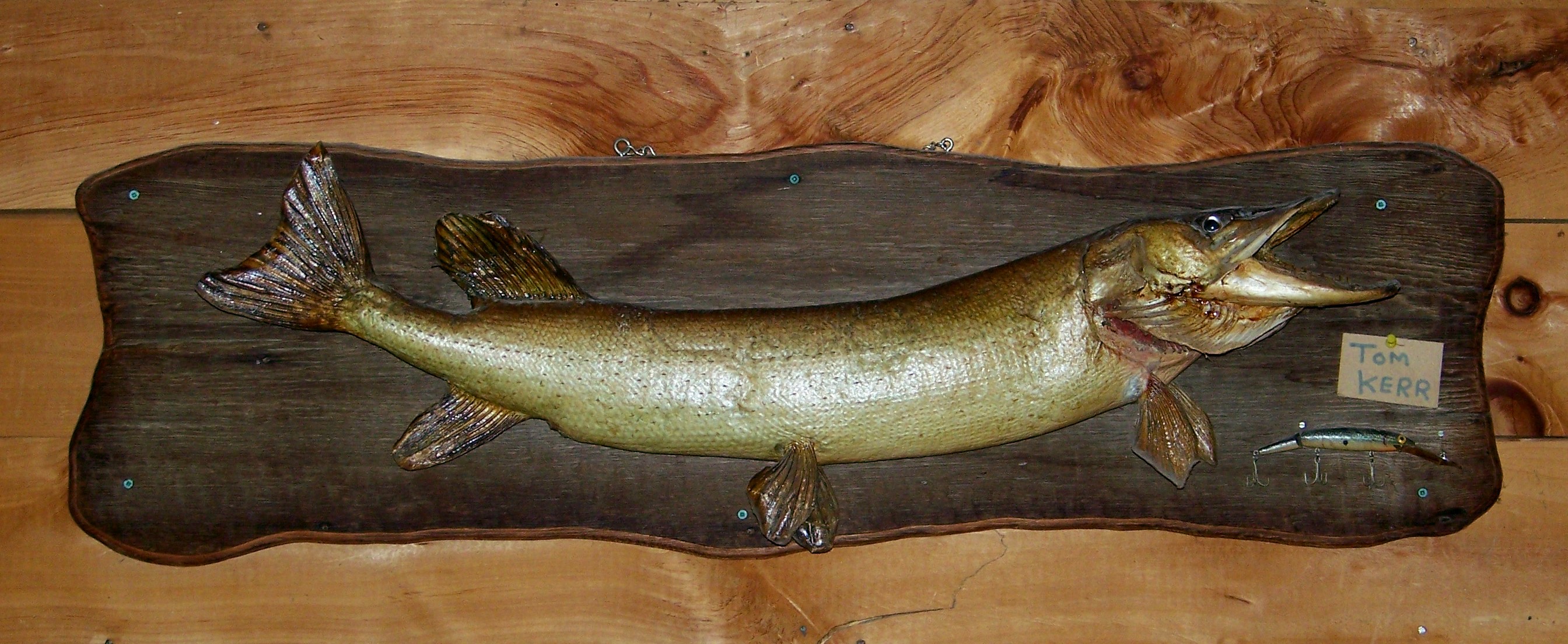The photograph showcases a mounted trophy fish displayed on an elegant wooden plaque, which is securely fastened to a wall of light brown, natural wood planks featuring visible knots and pronounced grain markings. The plaque is fixed with six screws, one in each corner and additional ones at the top and bottom. The fish, exhibiting signs of age, is curved with both its head and tail arched upwards. It boasts a striking dual-toned coloration, dark green on its dorsal side and fading to a lighter green and white on its belly. The fish has a large, open mouth reminiscent of a beak, and it features seven fins in total: one on its back and six on its underside, with the front fins appearing doubled. On the right side of the plaque, a small brown piece of paper is attached, displaying the name "Tom Kerr" in handwritten blue ink. Below this, a hanger featuring fish hooks and a simple fishing lure is also visible, suggesting these were used in catching the fish.